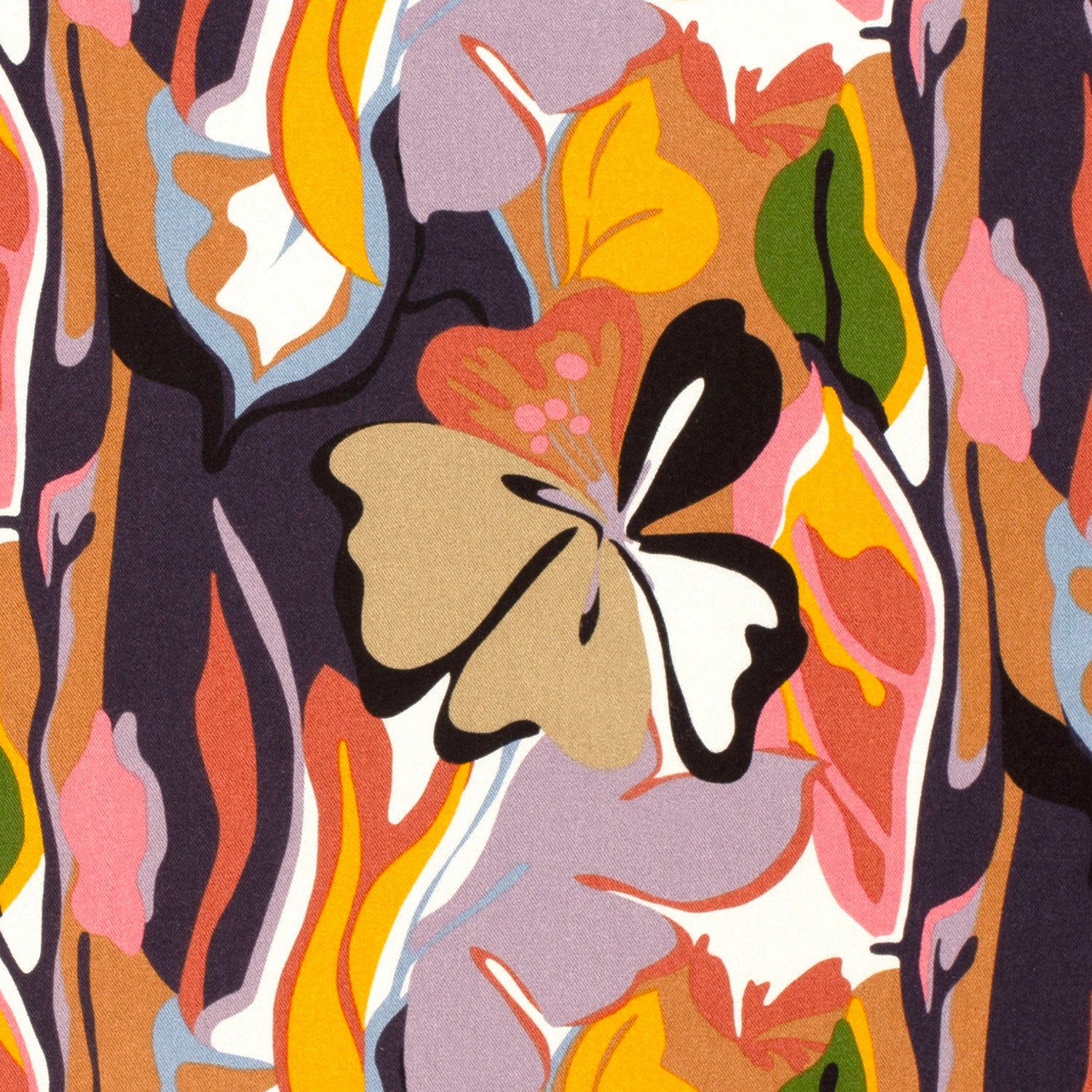The artwork, possibly a painting or fabric on canvas with a textured appearance, showcases a striking floral design. Central to the image is a prominent flower with an array of distinct petals: two beige outlined in black, two white also with black outlines, and a top petal that is tan merging into rosy hues, accented with gold and pink stamen dots. Surrounding this central flower is a colorful, slightly abstract background of swirling leaves and stems. The leaves and stems are depicted in a range of subdued yet diverse colors including dark purple, lavender, yellow, brown, green, pink, golden tans, and some areas outlined in black. These colors appear blended together, giving a sense of movement and fluidity to the overall piece. The combination of detailed central flower and the more muted, abstract background creates a visually captivating and pretty composition.